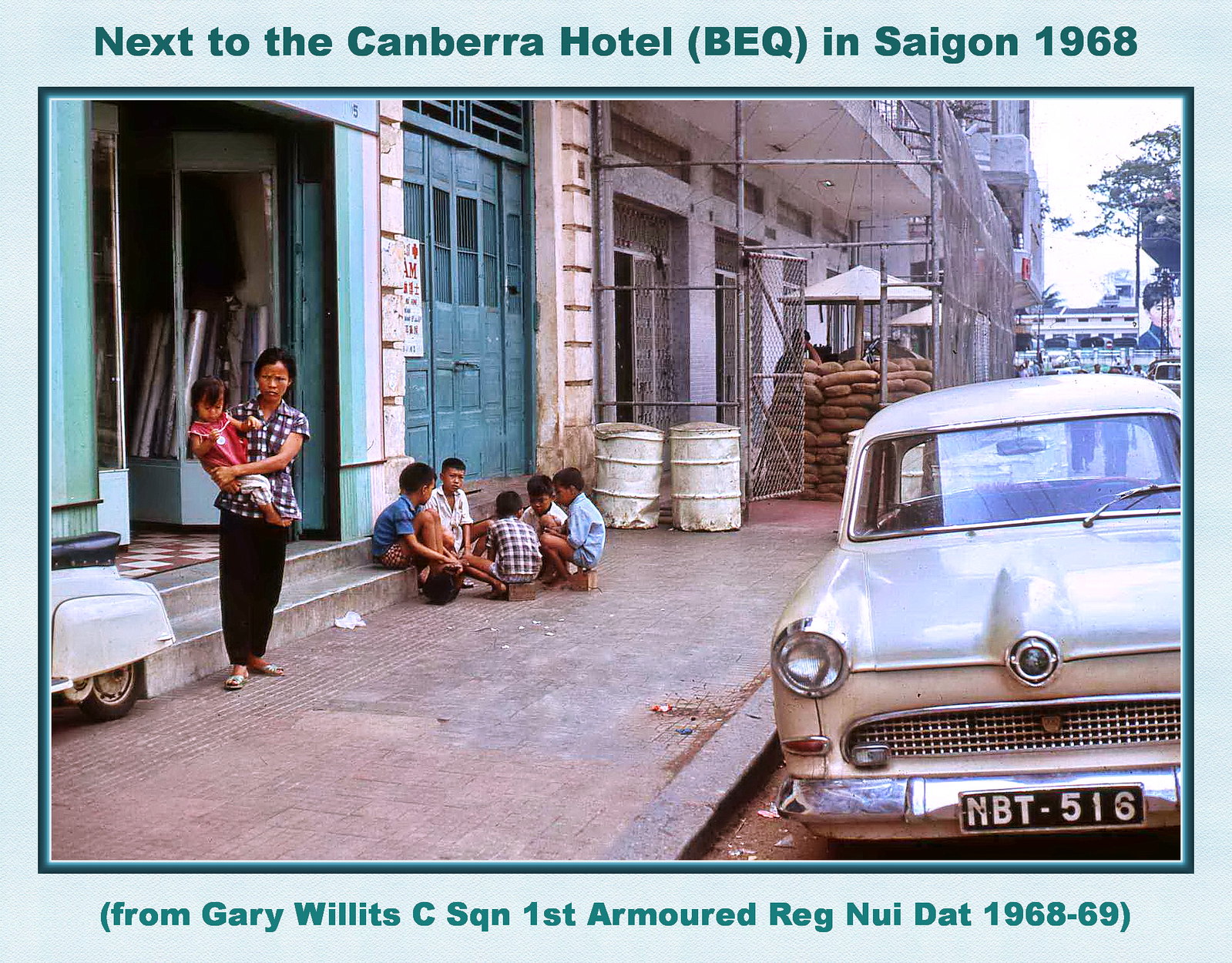This detailed photograph, bordered by a light blue outer edge with a dark blue inner frame, presents a vivid street view scene from Saigon, 1968. At the top of the frame, an inscription reads "Next to the Canberra Hotel, BEQ in Saigon, 1968," while the bottom indicates "From Gary Willits, CSQN, First Armored Reg, Nui Doat, 1968-69."

Central to the image is an Asian woman with a frowning, stern expression, holding a little girl in her arms, evidently displeased with being photographed. To their right, a group of Asian children sits on the ground in a circle, possibly engaged in play, and visible in the background are some open and closed doorways leading to various buildings. On the left side of the frame, part of a scooter can be seen, and to the right, an old-fashioned tan-colored car with a black license plate reading MBT-516 is parked by the curb. Further in the distance, there are additional buildings, some trees, and a construction area enclosed by a chain link fence with two white barrels by its entrance. The scene is a slice of life from a bustling urban sidewalk of 1960s Saigon.